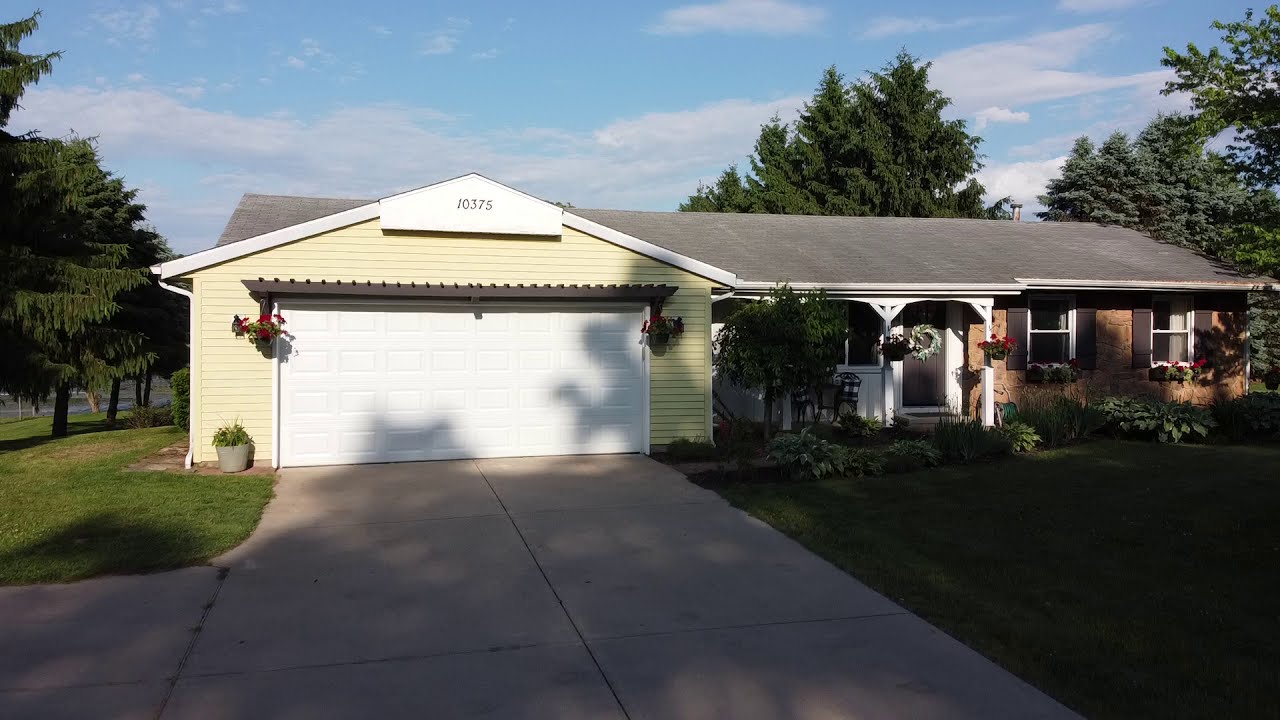This image showcases a charming, one-story ranch-style house with a meticulously manicured lawn and lush greenery. The house exterior combines wood siding and brick elements, featuring a light tan paneling and white trim. The garage, located on the left side of the house, has a spacious white door and a distinctive house number displayed above it. A sidewalk walkway lined with beautifully landscaped hosta plants leads up to the dark brown entrance door, which is adorned with a decorative wreath. In front, there's also a lovely crepe myrtle tree and hanging flower pots both over the garage and on the inviting small porch. The front yard is an expanse of vibrant green grass, complemented by evergreen trees around the house, adding a serene backdrop. The clean, shaded concrete driveway extends from the foreground up to the house, framing this picturesque suburban setting.